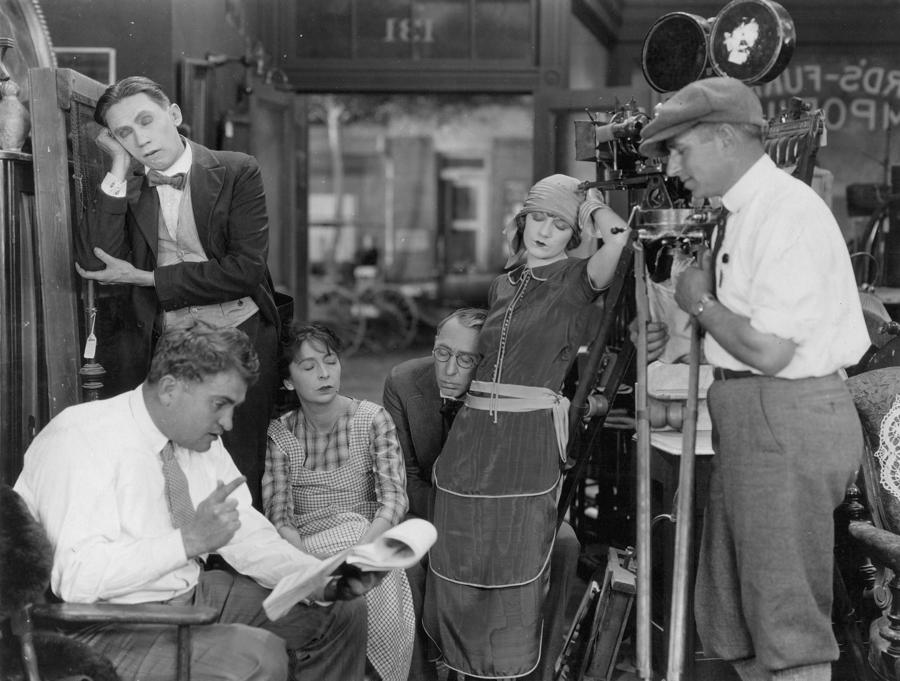In this black and white still frame from an old movie or TV show, set in what appears to be a 1920s-style interior room, six individuals are depicted, seemingly involved in some sort of broadcast. On the left, a man in a white button-down shirt, tie, and khaki-style pants sits holding a sheaf of papers or a notebook, appearing to read and gesture. Next to him, a woman in a long-sleeved top and apron-style dress is seated, her head resting in sleep against a man in a tuxedo who is also asleep and standing behind her, propping his head up with his hand. Adjacent to them is another man in a suit and glasses, also asleep and leaning against a standing woman. This woman, dressed in attire reminiscent of the 1920s including a hat and long dress, appears to be asleep while leaning against some furniture. Finally, another man in a white shirt with rolled-up sleeves, gray knickers, and a flat cap stands holding a piece of tall equipment, possibly a camera, which reaches up to his chin. Behind him is an old-fashioned motion picture camera, further anchoring the scene in its vintage film set environment. A notable detail is the presence of text in the photo, though it appears backwards and is difficult to read, adding to the aura of a snapshot capturing a moment of drowsy inactivity on a historic set.